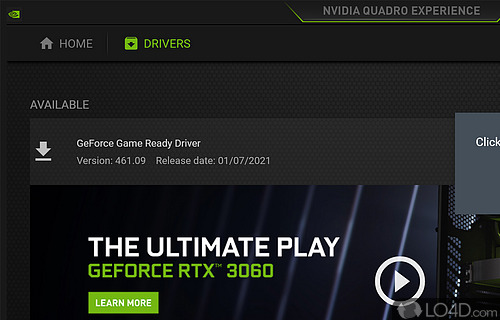This image appears to be a screenshot from the NVIDIA Quadro Experience website, characterized by its sleek black background accented with the company’s branded lime green. At the top of the page, there's a navigation menu starting with a home icon and the label "Home." To its right, the word "Drivers" is prominently displayed in the branded green, accompanied by a down arrow indicating a dropdown menu.

Beneath this navigation bar, a section labeled "Available" provides information about a driver update. The update prompts the user to download the latest GE Force Game Ready Driver. This section features a white download icon, which consists of a down arrow with a line underneath it, symbolizing the download action.

The driver version listed is 461.09, and it was released on January 7th, 2021. Underneath the driver download section, the text "THE ULTIMATE PLAY" is displayed in bold, white capital letters, adding a sense of importance and excitement. Directly beneath this, in capital letters and the signature green color, the text "GEFORCE RTX 3060" highlights the product focus, further enhancing the visual appeal and informational content of the page.